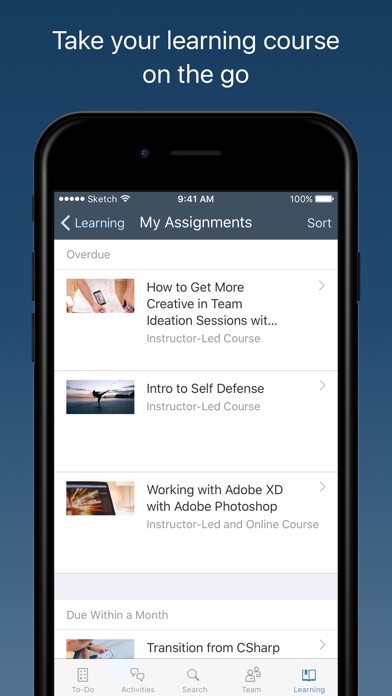This image appears to be an advertisement for a mobile learning platform. The background of the image features a clean grayish-blue gradient, creating a modern and professional look. At the top of the image, in bold white letters, the text reads, "Take your learning course on the go." Below this, a sleek black smartphone is prominently displayed, showcasing the app's interface.

The screen of the phone displays a learning dashboard with several course entries. The visible headings include "Learning," "My Assignments," and a sorting option. Notably, there is a section labeled "Overdue," highlighting assignments that need immediate attention.

The first course entry visible on the screen features a thumbnail image on the left beside the title, "How to Get More Creative in Team Ideation Sessions..." with an indication that it's an "Instructor-led Course." Following this, another course is listed with an image of a person stretching on a beach, titled "Intro to Self-Defense," also marked as an "Instructor-led Course."

Further down, the screen displays a course titled "Working with Adobe XD with Adobe Photoshop," indicating it's an "Instructor-led, Online Course." Additionally, there is a deadline reminder stating "Due within a month" and a course titled "Transition from C#." The final portion of the screen shows a partially visible image, cut off by the size of the phone's screen.

Overall, the ad effectively conveys the convenience and variety of courses available on this mobile learning platform, emphasizing its utility for on-the-go learning.